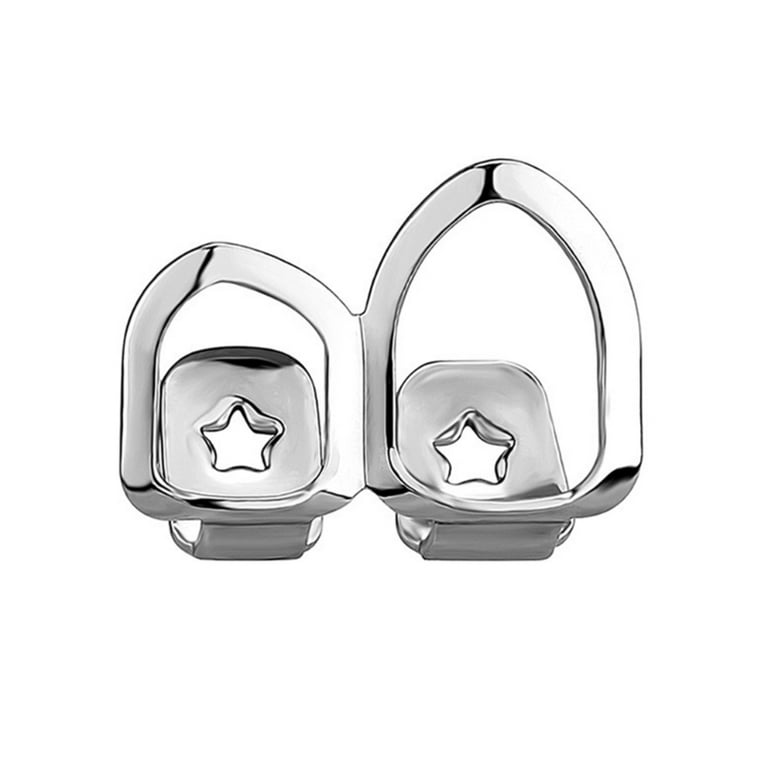The image is a color photograph in portrait orientation, featuring a chrome piece of jewelry, likely a two-section ear cuff or a similar object. The object is composed of two sections joined in the center, both sporting the same design. The section on the right is taller and wider, while the section on the left is shorter. The design includes two elliptical loops with an arched top and rounded edges at the bottom. These sections are connected by a silver rectangular bar, which extends downward and culminates in a flap that features a cutout of a star shape on both sides. The jewelry appears to float against a stark white background, emphasizing its reflective, shiny metal surface. The photo is a realistic product shot, showcasing the intricate details and craftsmanship of the jewelry.